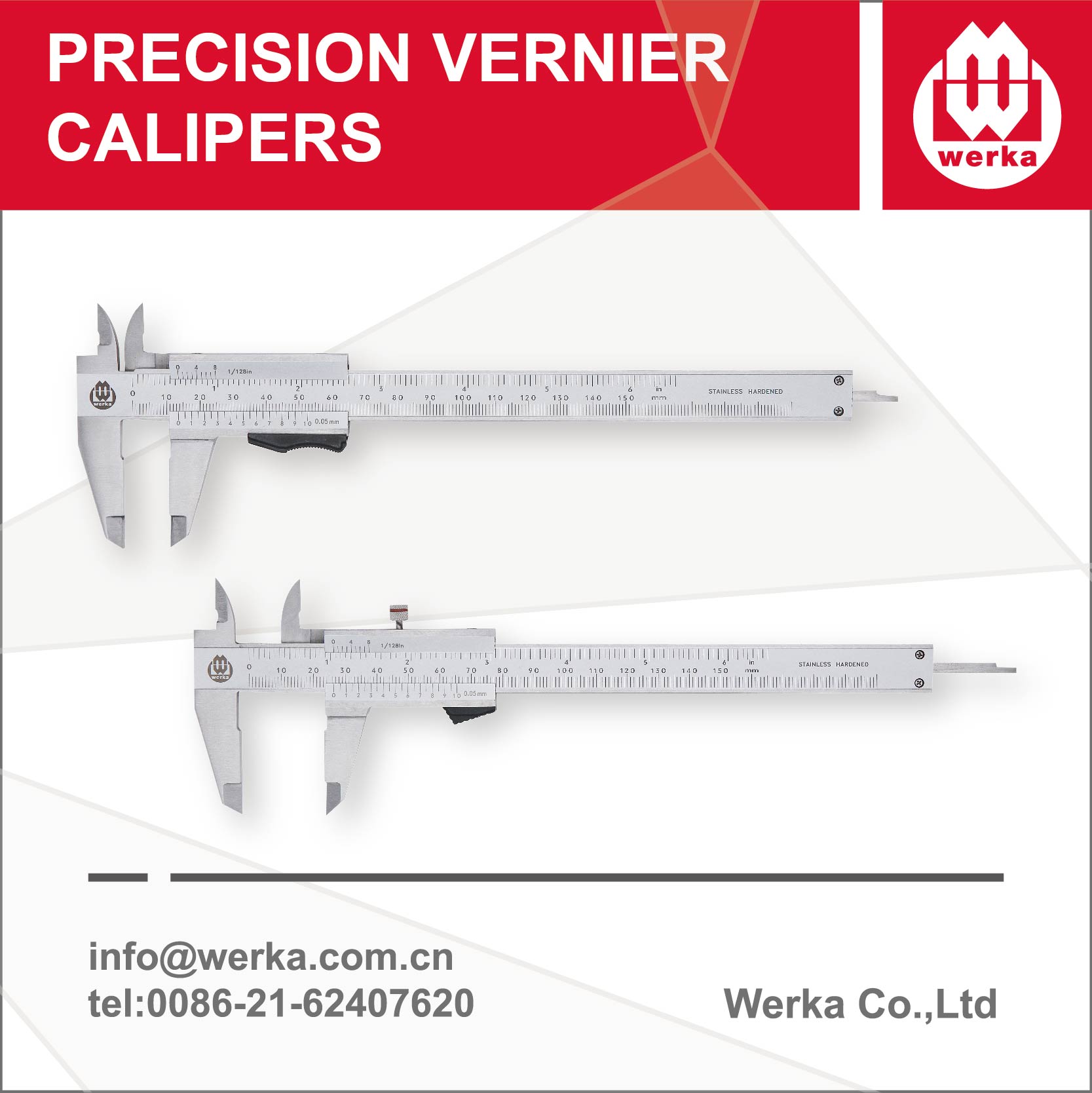The image prominently features precision Vernier calipers, highlighted by a red strip at the top with the text "Precision Vernier Calipers" in white. Positioned just below this header on the top right corner is the WERCA logo, which consists of a red square with a white circle containing an 'M' and a 'W', with "WERCA" noted in red text at the bottom of the logo. The central area of the image displays two calipers: the upper one with a smaller opening and the lower one with a larger opening, suggesting measurements of about half an inch and one inch respectively. Both calipers resemble rulers with claw-like measurement jaws and a screw to lock the measurement in place. Below the calipers, a black line separates the central image from the text details at the bottom. The background is primarily white with a very light gray triangle accentuating the layout. The bottom left corner lists the contact information, including the email address "info@WERCA.com.cn" and the telephone number "0086-21-62407620." The bottom right corner features the text "WERCA Co., Ltd."